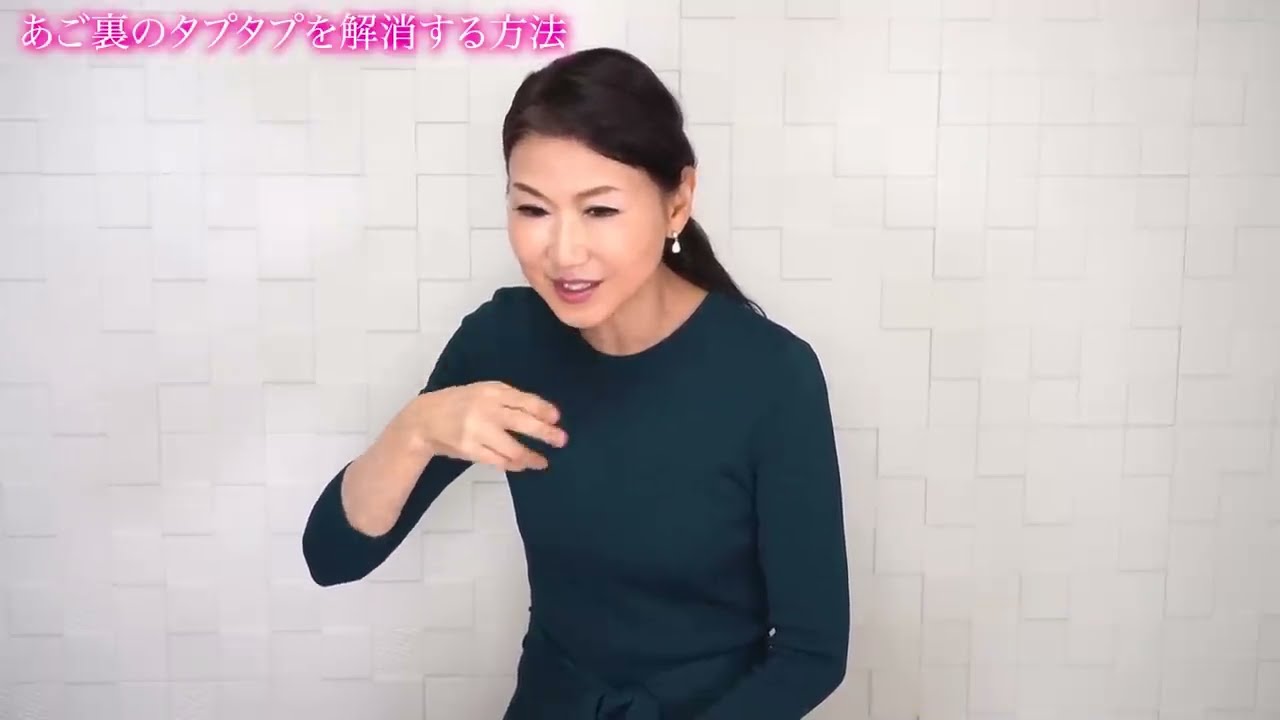This color photograph, likely a screenshot from a TV show, features an Asian woman, possibly in her 30s or 40s, who appears to be explaining something, suggesting she might be a teacher. The woman, pictured from the waist up, has long black hair pulled into a low ponytail and is wearing noticeable makeup including red lipstick. She is dressed in a form-fitted, dark-colored long-sleeve top, with descriptions varying between black, dark green, and grayish-blue. Dangling pearl-like earrings add a touch of elegance to her appearance.

She is posed against a geometrical white brick wall with a stair-step pattern. In the top left corner, vibrant text, believed to be in Mandarin or Japanese, is visible in bright magenta outlined with white. The woman has her right hand raised, possibly indicating she is about to eat something or making a gesture to emphasize her speech, while her left hand is not visible. She is smiling partially and looking slightly downward, adding a calm and engaging demeanor to her explanation.